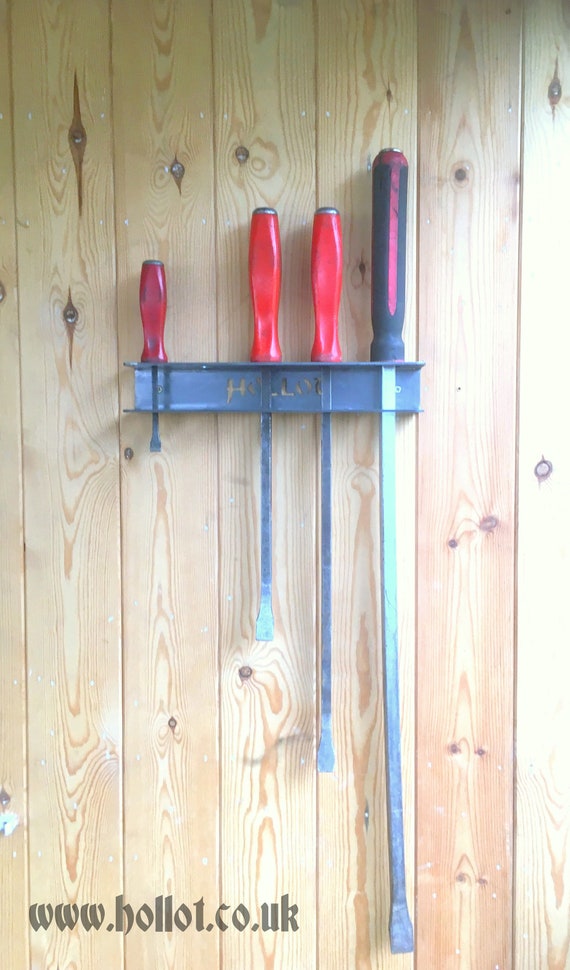This is a color photograph featuring a vertical tool rack specifically designed for screwdrivers, mounted on a wooden wall composed of light-colored slabs with darker brown grain and prominent dark brown knots. There are visible silver nail heads in the wood. The metal bracket, resembling a small I-beam, is painted blue and is screwed into the wall. It has a series of holes in which four screwdrivers are neatly placed. The leftmost screwdriver is the shortest, with a red handle, and they progressively increase in size towards the right. The three screwdrivers on the left share the same shiny red handles, while the rightmost one features a dark gray rubbery handle with a red area near the tip and a red streak along the side. All the screwdrivers are of the flathead variety. The rightmost screwdriver is exceptionally long, extending to the bottom of the photograph. A semi-transparent red watermark reading "www.hollett.co.uk" is visible in the lower left corner of the image.